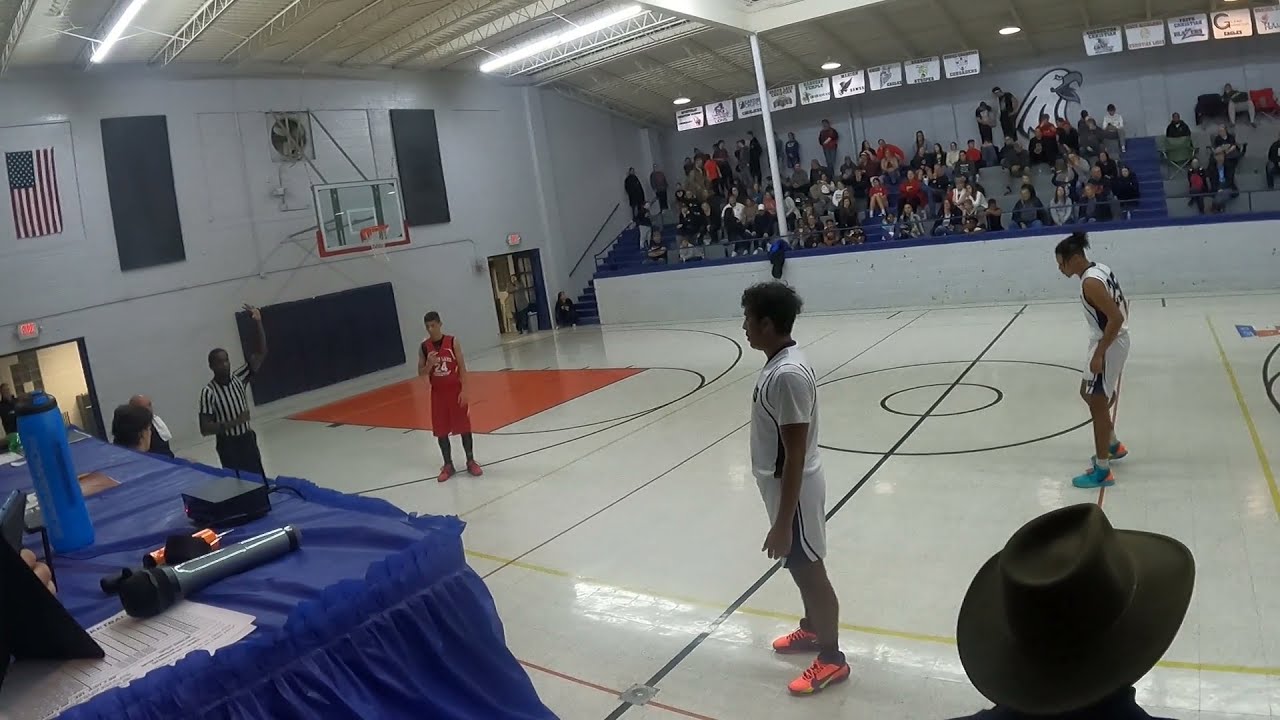The image depicts the inside of a predominantly white basketball court, where a game seems paused with the players awaiting the next move. In the bottom left corner stands the announcer's table, covered in a blue vinyl tablecloth, equipped with a microphone, papers, and a thermos. Nearby, a referee, clad in standard black slacks and a black-and-white striped top, raises his left arm in the air. Adjacent to him is a young male player in a red basketball uniform. To the right, another young player in a white jersey faces the referee, and farther back, yet another player in a white uniform stands. Behind the scene, an American flag adorns the wall and above it, a ventilation fan hovers over the basketball backboard and hoop. The gym’s bleachers are densely populated with fans, possibly around a hundred, with a black and white eagle head mascot painted on the wall behind them. On the right, a person wearing a cowboy hat is partially visible. The atmosphere is one of anticipation, as everyone seems poised for the game to resume.